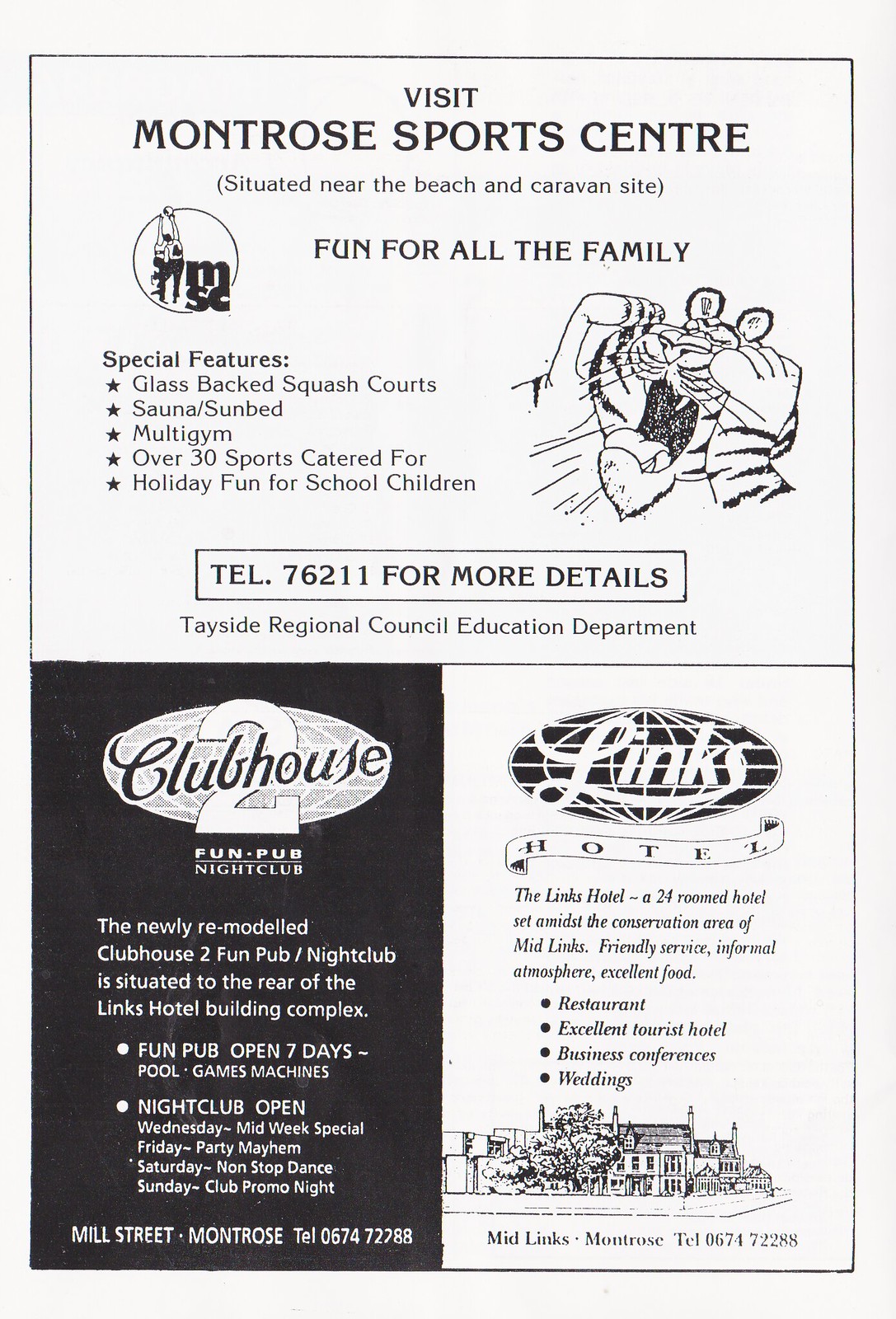This is a detailed ad page from a magazine or newspaper, divided into three sections. The top section prominently features an advertisement for Montrose Sports Center, which has a white background and black lettering. It reads, "Visit Montrose Sports Center," and mentions that it is "situated near the beach and caravan site" with the phrase "Fun for all the family" emphasized below. Next to the text, there's a black-and-white cartoon drawing of a tiger with its mouth open and hands up to its mouth, as if yelling "Fun for all the family." The ad highlights several special features of the sports center, including glass-backed squash courts, saunas, sunbeds, a multi-gym, and facilities catering to over 30 sports. It also offers holiday fun for school children. For more details, a telephone number is provided along with a note indicating the Tayside Regional Council Education Department.

Below this, in the lower section, there are two vertical advertisements side by side. On the left, there is an ad for Clubhouse 2, a fun pub nightclub. The rectangular ad, set against a black background with white text, notes that the Clubhouse 2 is newly remodeled and located in the rear of the Lynx Hotel building complex. It lists the fun pub as being open seven days, featuring pool games and machines, with the nightclub open Wednesday, Friday, Saturday, and Sunday for various themed nights.

On the right, there is an advertisement for the Lynx Hotel, which features a line drawing of a resort and a logo. It highlights the hotel's 24 rooms set amidst a conservation area of Mid Links, promoting its friendly service, informal atmosphere, excellent food, and suitability for tourists, business conferences, and weddings. A contact phone number is also provided at the bottom of the ad.